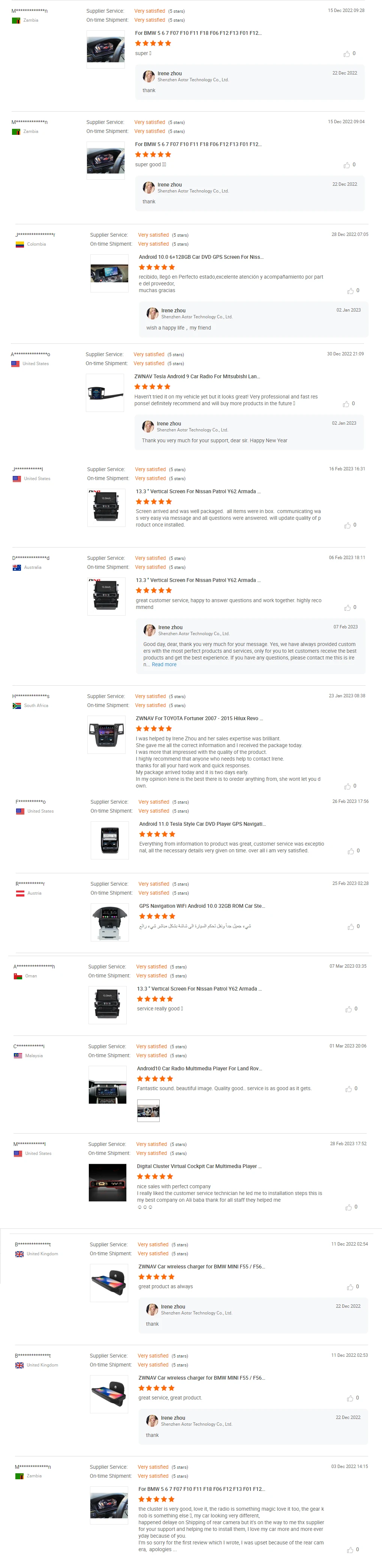The image showcases a structured layout with four distinct columns. The first column features a horizontal bar at the top and a space presumably for an emoji or an icon, followed by a smaller line that seems to be for additional input. 

Adjacent to this, the second column displays a larger image along with a set of star ratings, all consistently showing five orange stars across the items. The detailed star ratings indicate a visual representation of quality or approval.

The third column, positioned at the far end of each row, appears to be a text column, although the print is too small to decipher clearly. Each entry in this column contains five lines of faint text, making it difficult to read the specifics.

Overall, the structure repeats for a total of 15 rows, each showcasing the same uniform elements: a bar in the first column, a large image with five orange stars in the second, and five lines of text in the third. The consistent layout suggests these are individual advertisements or listings of some sort.